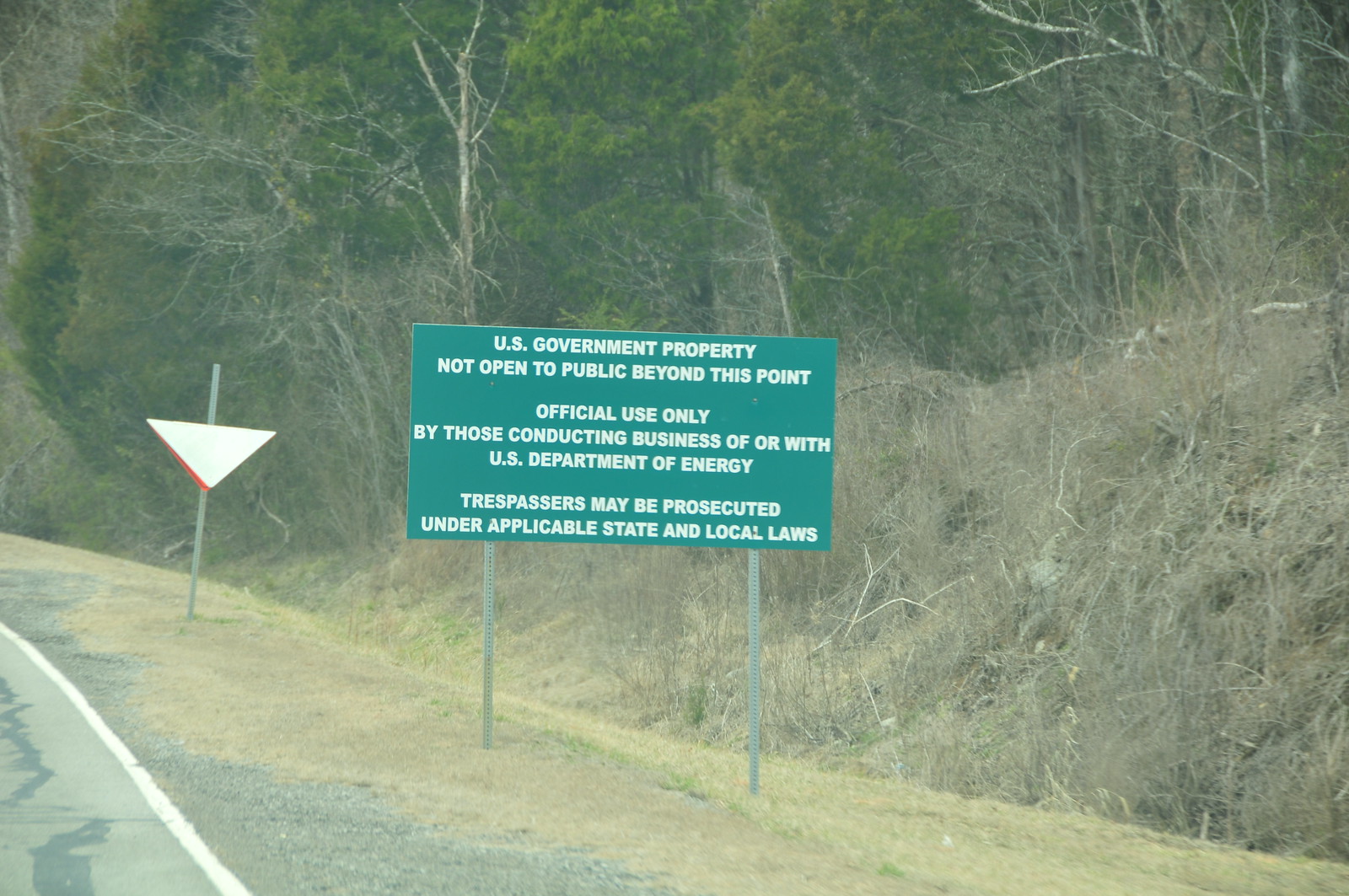The image features a prominent green sign, indicating a restricted area under the jurisdiction of the U.S. Department of Energy. The sign reads: "U.S. Government Property. Not Open to the Public Beyond This Point. Official Use Only by Those Conducting Business of or with U.S. Department of Energy. Trespassers May Be Prosecuted Under Applicable State and Local Laws."

To the right side of the sign, there are lush green trees, adding a natural barrier. The bottom right corner of the image displays patches of brown earth or underbrush. On the left side, a railway track runs parallel to the scene, and near it, a white, black, or possibly red object lies folded on the ground.